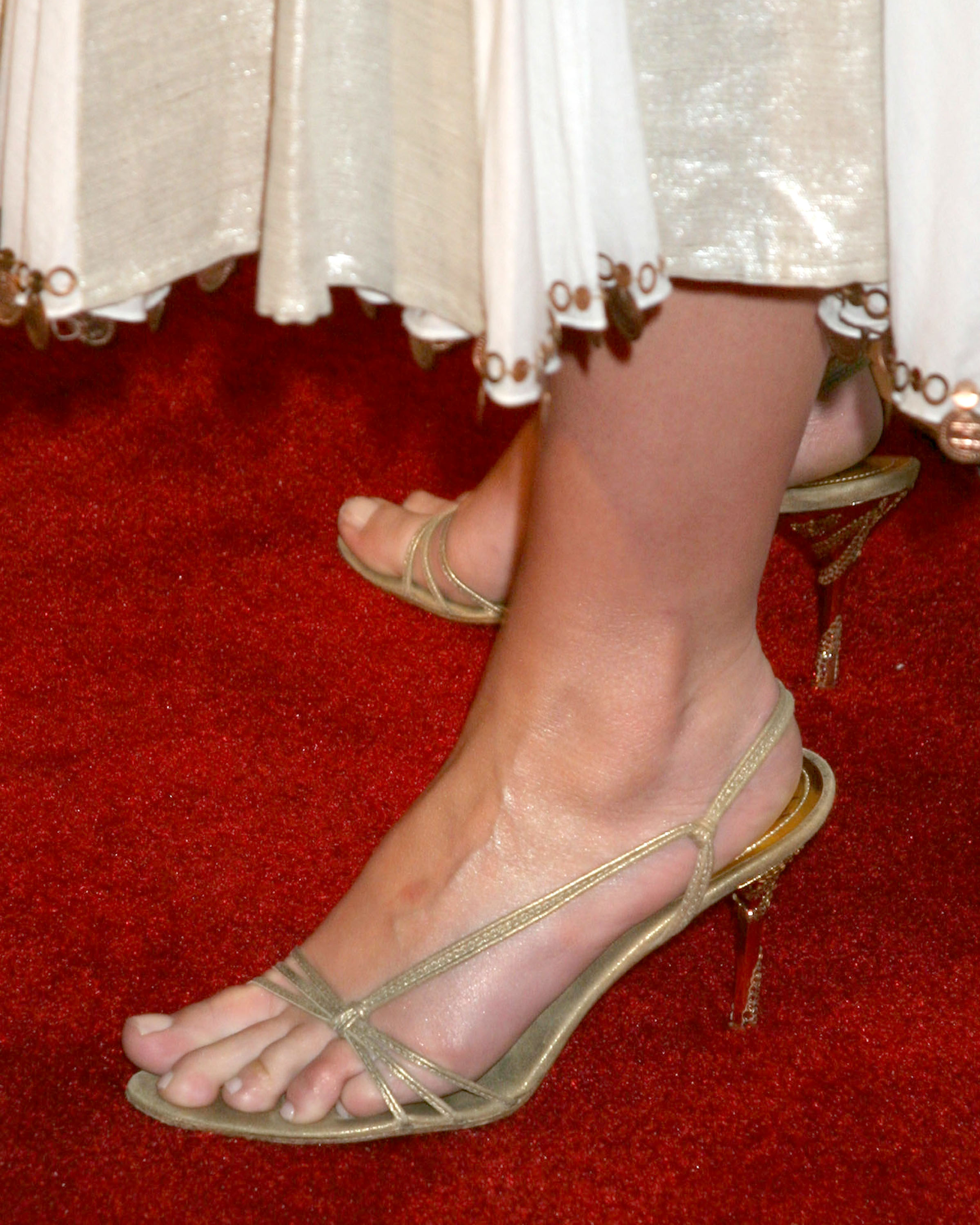The image captures an elegant scene focused on a woman's feet adorned in stylish footwear. The woman is wearing gold heels with thin, strappy designs that include hints of red on the bottom and gold trim. Her feet, one prominently in the foreground and the other slightly behind, are seen standing on a luxurious, fluffed red carpet with a stark red hue. The woman's attire complements her footwear, featuring a shimmering, silvery-white dress with bronze and golden accents, including delicate dangling accessories. The hem of the dress, detailed with sequins, extends across the top of the photograph, adding a touch of glamour to the overall composition.